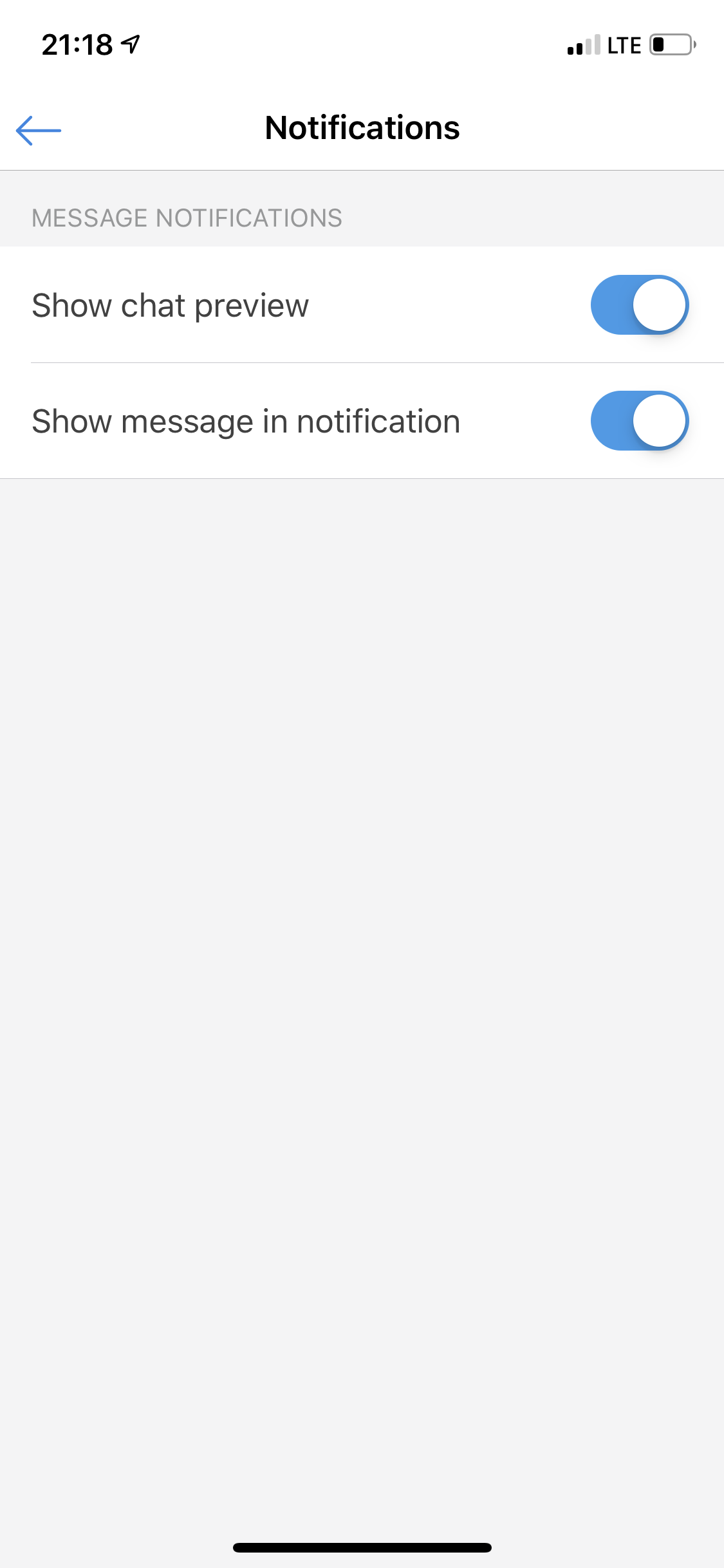This image is a screenshot of a smartphone's notification settings screen taken at 21:18. In the top left corner, there is a small paper plane icon, while the top right corner displays the phone's signal strength with four bars and an LTE indicator. The battery icon shows a nearly depleted battery.

Below the time, there is a section labeled "Notifications" featuring a left-pointing blue arrow. Beneath this is a gray line followed by a gray box titled "Message notifications" in light gray text.

Next, there is a white section labeled "Show chat preview" with a toggle switch that is turned on, indicated by the blue color. Another option titled "Show message notifications" also has its toggle switch turned on, showing blue. The bottom part of the screen contains a rectangular gray space, followed by a horizontal black line at the very bottom, with no additional content visible.